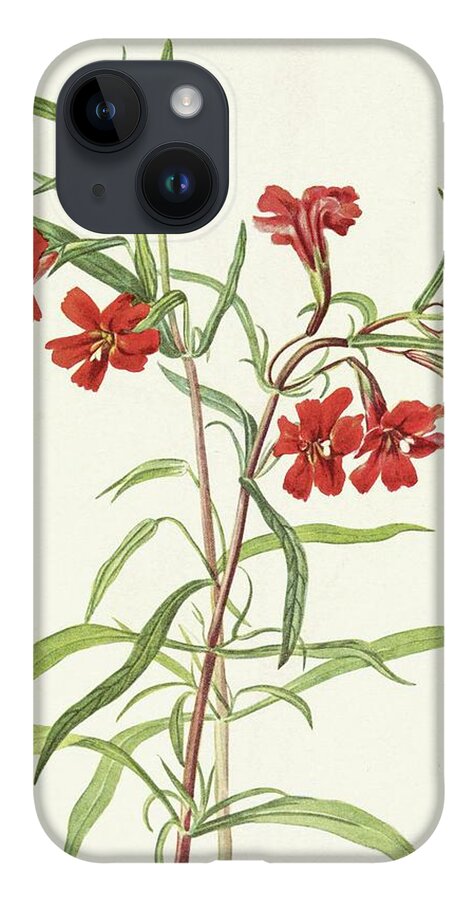The image depicts the back of an iPhone encased in a protective cover with a predominantly white background. The cover features a detailed floral design, highlighting intricate vine-like structures. The stems, which are a rich burgundy or brown, intersect and support elongated, slender green leaves. Scattered throughout the vines are small, red flowers with slightly wavy, rectangular petals, and subtle hints of yellow at their centers. Four complete flowers and a portion of a fifth flower are visible. In the upper left corner of the image, the iPhone's camera array is prominently displayed, showcasing two large black lens circles alongside a smaller light dot. The phone itself appears to be a modern, dark gray iPhone model. Overall, the case presents a charming, botanical aesthetic while maintaining a simple and elegant design.